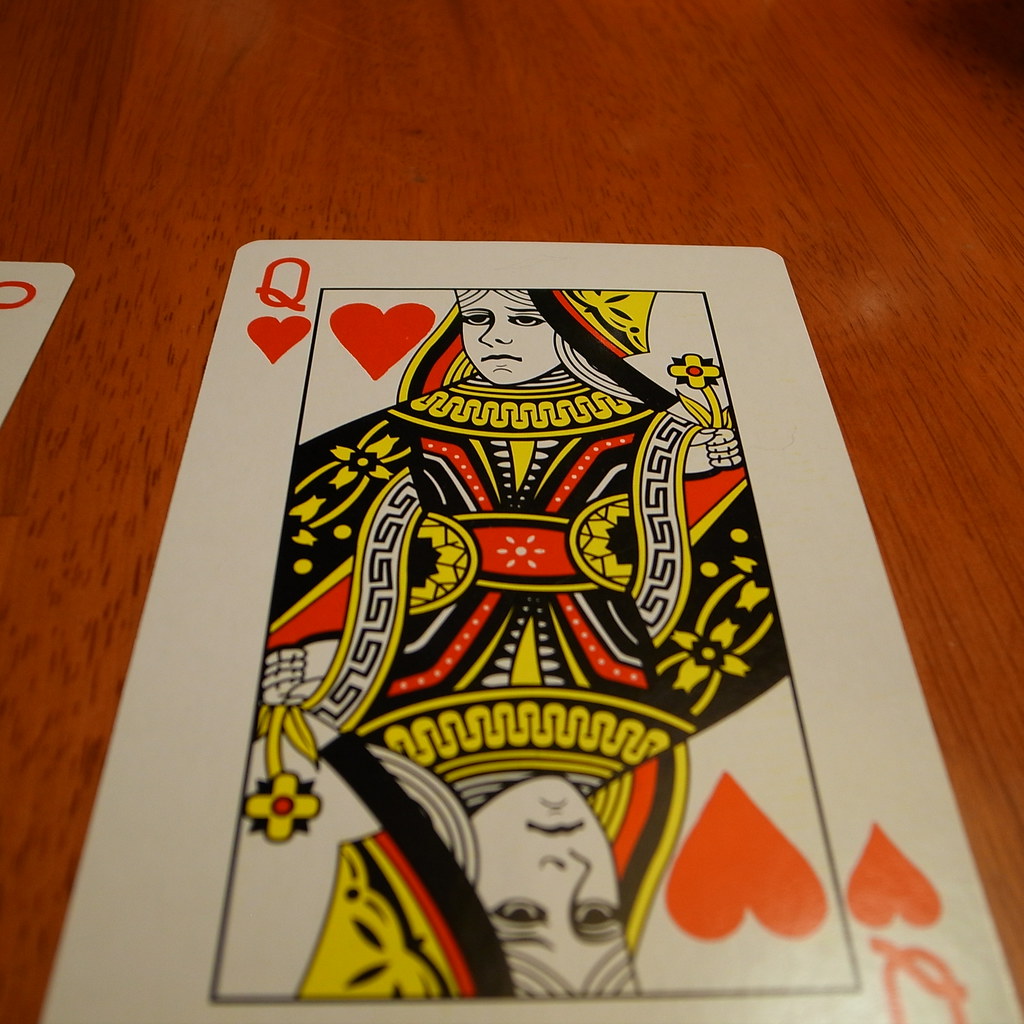This is a detailed close-up image of the Queen of Hearts playing card set against a wooden surface. The card is angled so that it appears larger at the bottom, gradually tapering off toward the top. The Queen of Hearts features a rounded border and showcases the letter "Q" in both the top left and bottom right corners, each accompanied by a heart symbol below. The design of the card is mirrored, ensuring that the Queen and her distinguishing features remain upright whether the card is flipped or not. Encased within a thin black border, the Queen's face is rendered in black and white, while her regal attire is vibrantly colored in black, yellow, red, and white. Her flowing clothing is elaborately decorated with intricate patterns extending from her neck down to her waist, at which point the image flips to mirror itself. The Queen wears a sullen expression, adding intrigue to her already intricate design. The overall composition, with its meticulous detailing and use of mirrored imagery, makes for a captivating visual presentation.